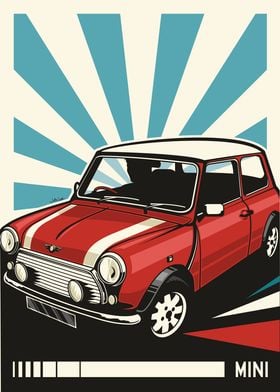The digital art piece depicted is of a bright red Mini Cooper minivan, centrally positioned in a vertically oriented, rectangular frame. The Mini Cooper features distinctive styling with dual white stripes running from the windshield down to the front headlights, and a completely white roof. The car's rims are rendered in white, matching the color scheme of the roof and stripes. The artwork captures the vehicle from an angle that predominantly shows the left side, including part of the front left and back left tires. The car's grill integrates two headlights and parking lights.

The background is an off-white or cream color, decorated with blue and turquoise radial lines emanating outward from the car, contributing to a starburst effect in the top half of the image. The bottom portion of the frame is detailed with a horizontal white bar, within which "MINI" is prominently displayed in capitalized white letters on the right side. This section also includes subtle hues of black, blue, and red. Overall, the image is crisp, vibrant, and well-lit, emphasizing the bright and lively presentation of the iconic Mini Cooper.